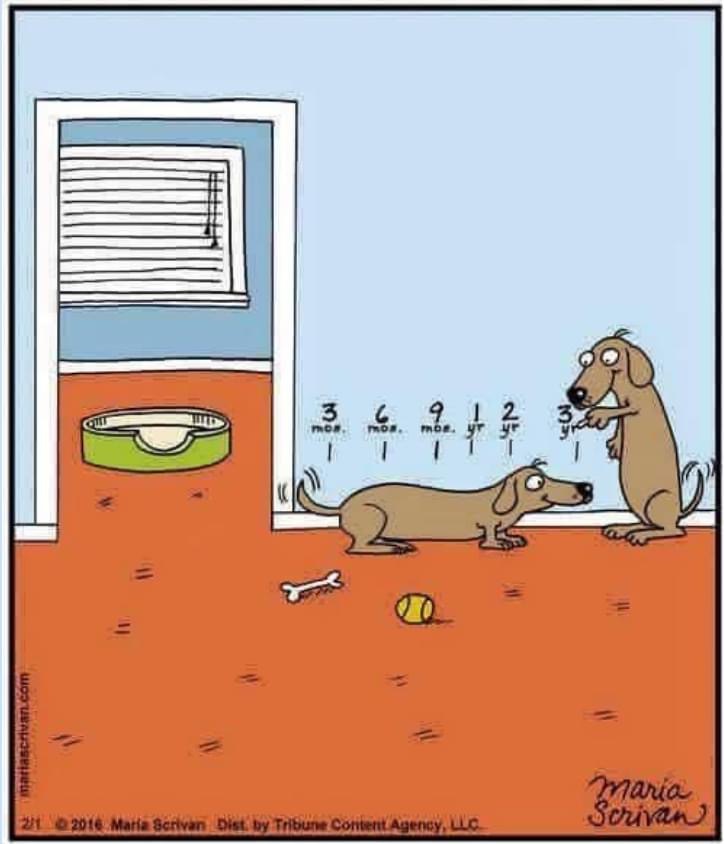This detailed cartoon panel by Maria Scriven, copyrighted in 2016 and distributed by Tribune Content Agency, features two brown dachshunds in a domestic setting. The background depicts a light blue wall adorned with measurements, marking the growth of the younger dog. The vertical marking system reads "3 months, 6 months, 9 months, 1 year, 2 years, 3 years," indicating the dog's length rather than height, which is humorously akin to how humans measure height on a doorframe.

The scene shows one dog standing upright, using a marker to measure the other dog's length against the wall, with a pleased parental expression. This playful mimicry is set in a house with a brown checkered carpet, a green dog bed, a white-framed window with closed blinds, and scattered toys, including a green tennis ball and a white bone. The ambiance is warm and domestic, emphasizing the familial bond and growth milestones familiar to human experiences but adapted amusingly to canine context. The artist's signature and copyright details, "Maria Scriven, 2016," are clearly visible at the bottom right of the panel.